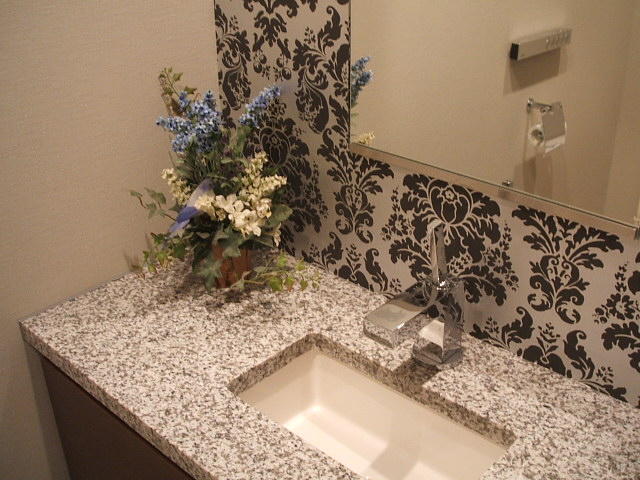The photo captures an elegantly designed bathroom taken from an overhead perspective of a single sink. The sink features a longer rectangular countertop, likely made from white granite adorned with intricate brown speckles. The sink itself is small, rectangular, and fairly deep, complemented by an angular, square faucet with a distinctive vertical pull-down feature. 

The wall behind the sink is decorated with striking brown and white floral wallpaper, showcasing a budding flower pattern with intricate leaves and curly cues that cascade outwards, enhancing the room's elegant aesthetic. On the left corner of the countertop, an arrangement of faux flowers in blue, white, and green hues adds a touch of freshness. The cabinet beneath the sink is painted in a sophisticated dark gray, while the adjacent wall on the left is a neutral white, providing a calming backdrop to the vibrant floral designs.